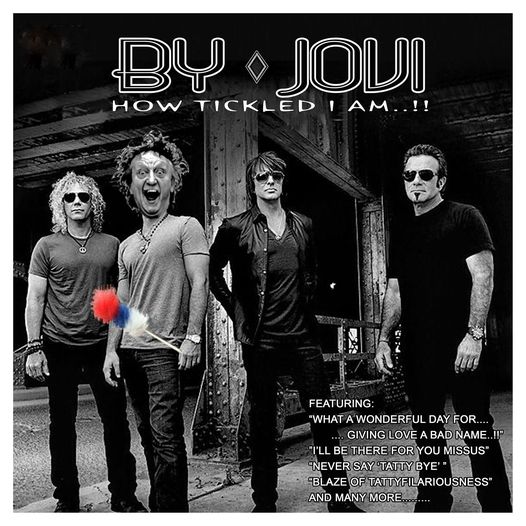The image is a humorous spoof of a Bon Jovi album cover titled "By Jovi: How Tickled I Am." It features a black and white photograph of four people, reminiscent of the original members of Bon Jovi, standing under an overpass or railway. The men, dressed predominantly in black and gray and wearing sunglasses, are lined up from left to right. Notably, the second man from the left stands out with his mouth open, messy hair, and holding a red, white, and blue feather duster.

The text "By Jovi" is prominently displayed at the top in white lettering, followed by the secondary title, "How Tickled I Am." In the lower right corner, in small white text, are spoofed versions of Bon Jovi song titles: "What a Wonderful Day," "Giving Love Bad Name," "I'll Be There for You, Mrs.," "Never Tatty Bye," and "Blaze of Tattie Filariousness," along with various other humorous adaptations. The combination of the visual setup and play on song titles creates a comedic homage to the band's iconic style.